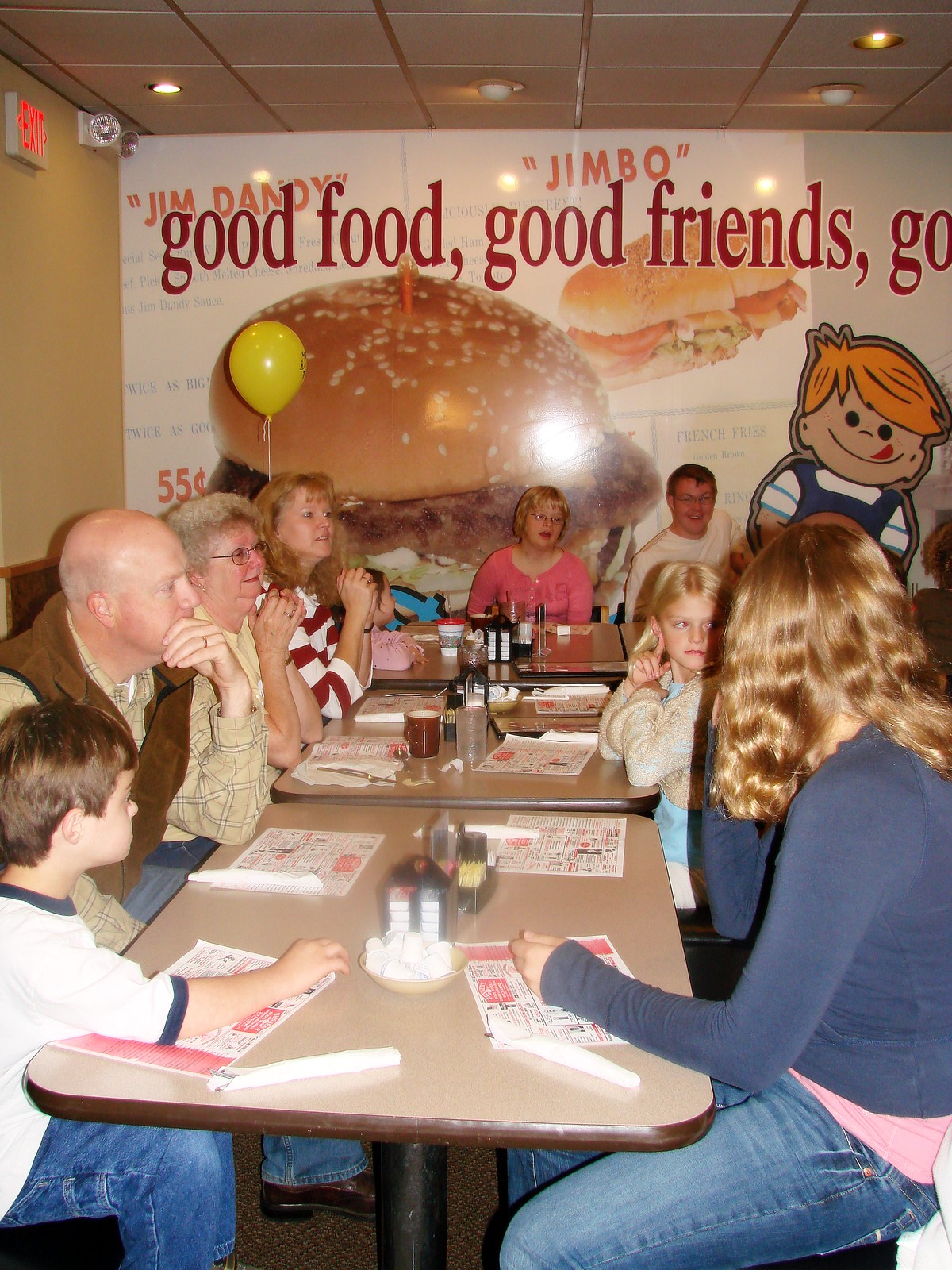In this photo, a diverse family group of around 10 to 12 people, including children, middle-aged adults, and senior citizens, gathers at a diner named Jimbo's, possibly celebrating a birthday as evidenced by a yellow balloon. The diners are seated at three to four tables covered in paper plates and menus, with silverware wrapped in white napkins. The focal point in the background features an advertisement displaying assorted hamburgers and sandwiches, as well as a cartoon image of a little boy with his tongue sticking out, and a nostalgic sign that reads "Jim Dandy's Jimbo - good food, good friends" along with "55 cents off", indicating the photo might be from an older era. The family's attention is directed towards the right side of the image, which is cut off, leaving what's captivating them to the imagination. The setting, filled with browns, tans, pinks, yellows, oranges, dark blues, and beige tones, creates a warm and nostalgic ambiance inside the diner.